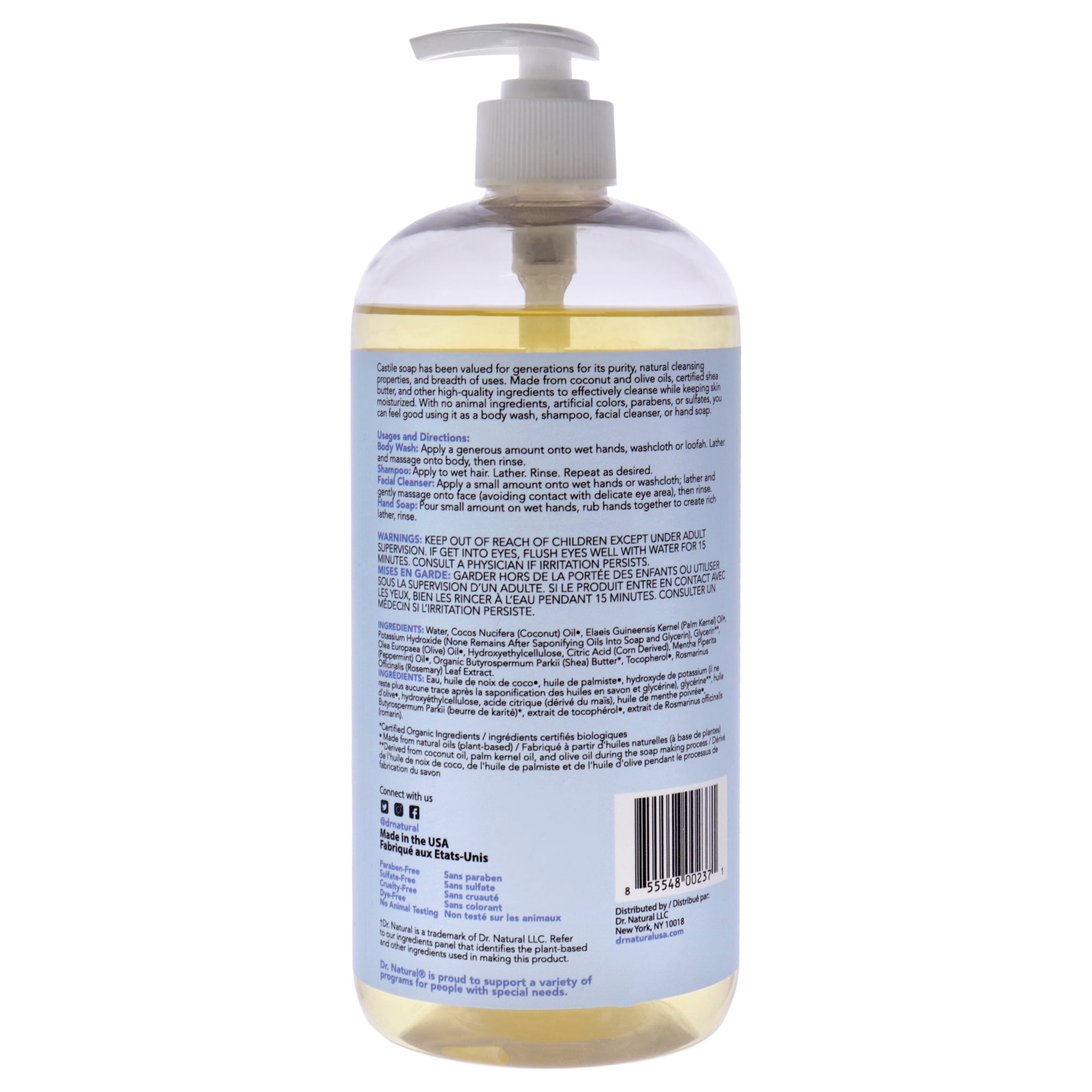The image showcases a round bottle with a white pump dispenser cap, containing a light yellow liquid. The bottle features a prominent light blue label on the front that reads "Castle Soap." This soap, highlighting its versatility and purity, is lauded for its natural cleansing properties, made from ingredients like coconut and olive oils, certified shea butter, and other high-quality components. The label describes the soap's effectiveness in moisturizing the skin while also being free of animal ingredients, artificial colors, parabens, and sulfates, making it suitable for use as a body wash, shampoo, facial cleanser, or hand soap. At the bottom of the label, there are sections dedicated to uses and directions, warnings, and ingredients, with a barcode on the bottom right corner. The bottle also mentions that it is made in the USA by Dr. Natural, LLC, inviting consumers to connect with the brand. The back of the label, visible but partially obscured and hard to read, curves around the bottle, containing further instructions and smaller print.